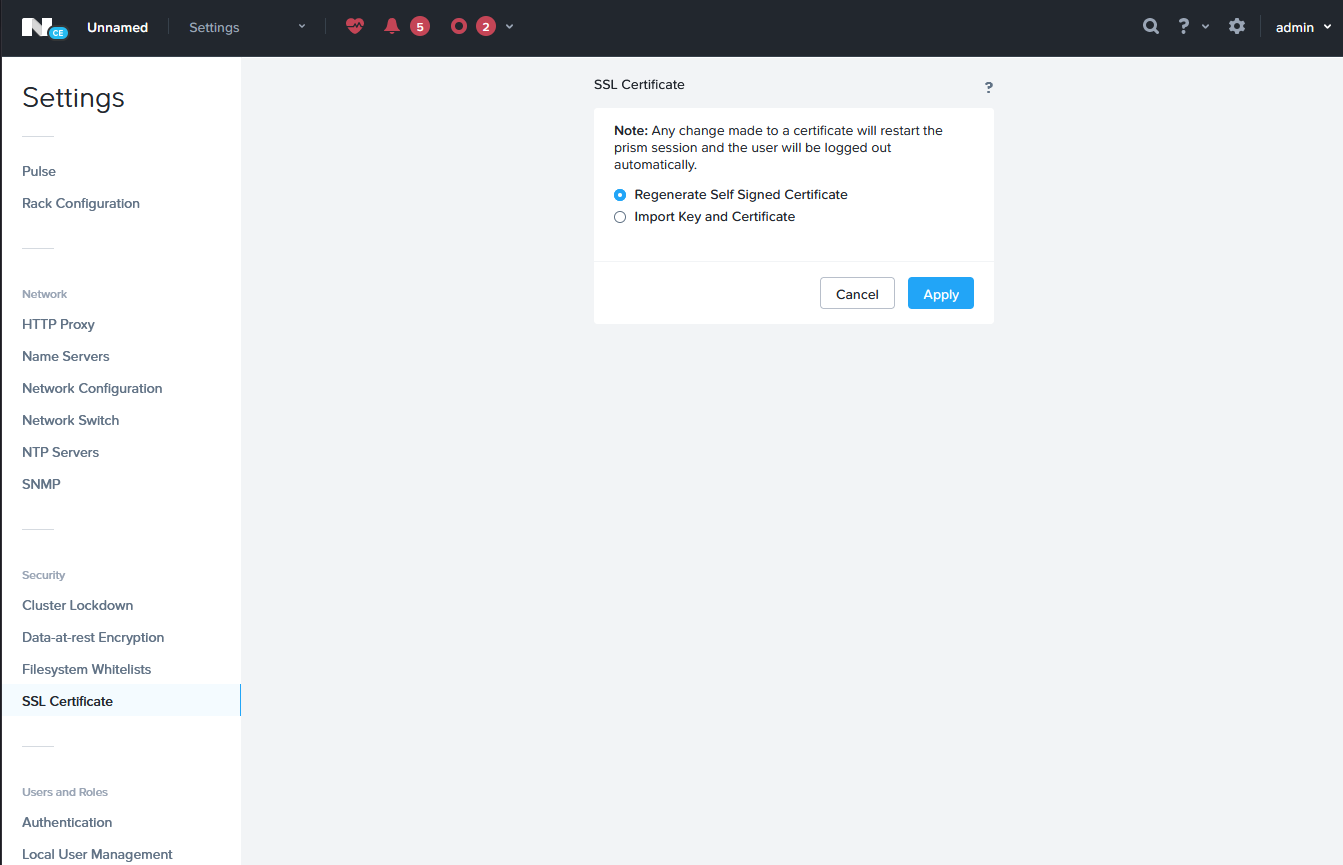This screenshot depicts a website open to the settings page. At the top, there's a black navigation bar featuring white text and several red icons, including a heart and a bell. The bar also includes icons for a question mark, a magnifying glass, and a settings gear.

In the main section, prominent black text reads "SSL Certificate." A white pop-up with black text warns, "Note, any change made to a certificate will restart the PRISM session and the user will be logged out automatically."

Below the warning, there are two selectable options: "Regenerate Self-Signed Certificate" and "Import Key and Certificate," each accompanied by a radio button. At the bottom of the pop-up, a gray "Cancel" button, styled with white text, and a blue "Apply" button, also with white text, offer user interactions.

On the left sidebar, black text labels several settings categories, including "HTTP Proxy," "NTP Servers," and "Security."